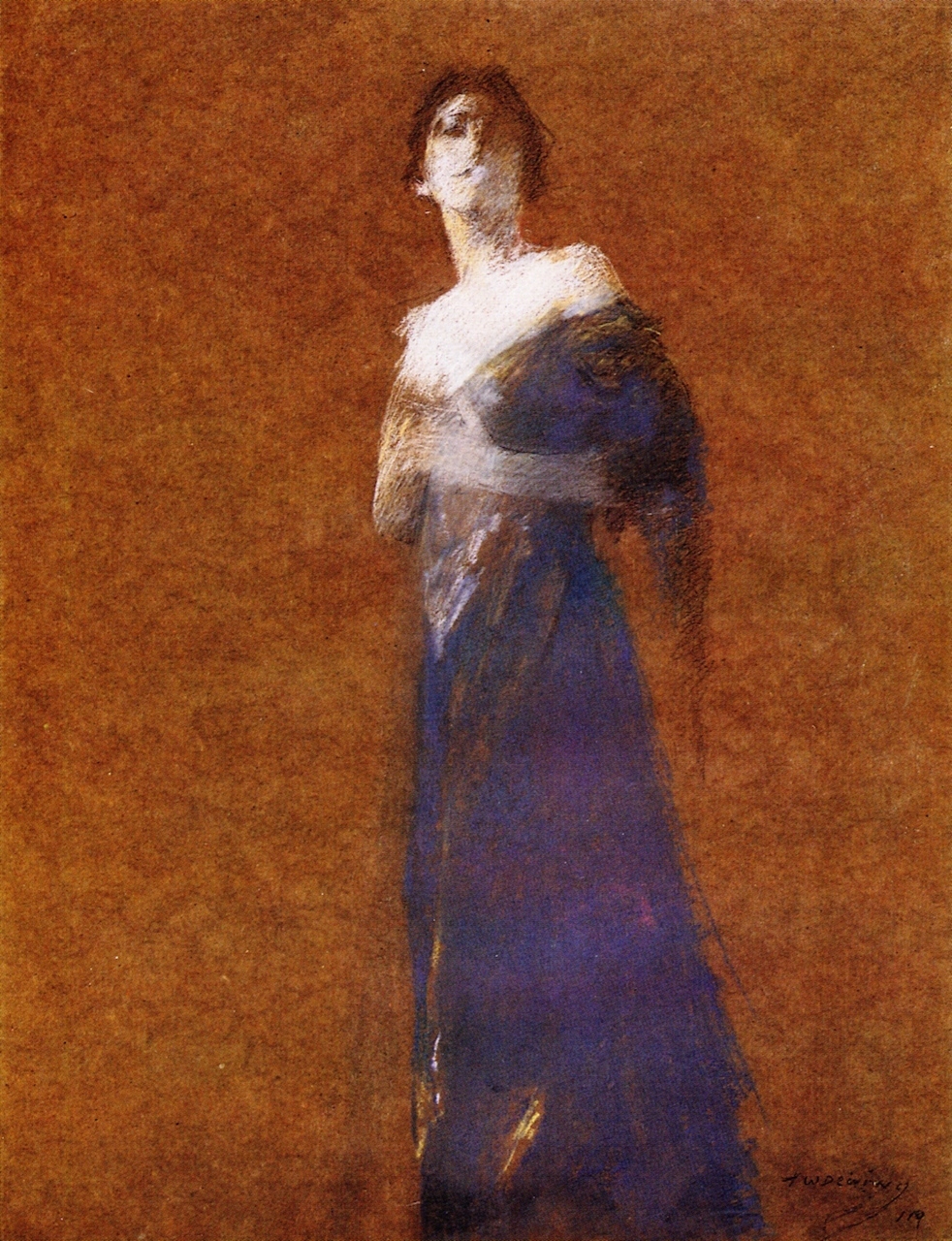This painting presents a figure of a woman standing in an ethereal and blurry manner, immersed in a predominantly deep, mottled brown background, with shades akin to dark burnt red and rusty orange. The woman, the painting’s sole focus, is depicted wearing an elegant off-the-shoulder dress that blends shades of blue and hints of gold or purple, draping from her chest down to the ground, leaving the upper part of her chest exposed. Her dark hair is pulled back, and her complexion is a stark ghostly white, contrasting dramatically with the muted, shadowy details of her indistinct facial features. She stands with her body somewhat turned to her right, the left of the image, with her arms faintly up against her chest in a pose that suggests both grace and incompletion, as one arm fades into a splotchy, translucent line. The perspective of the painting is slightly below her, adding a subtle sense of elevation to her stance. At the bottom of the painting, there's an artist’s signature and the number “119,” although it's difficult to decipher clearly due to its small, blurred script.